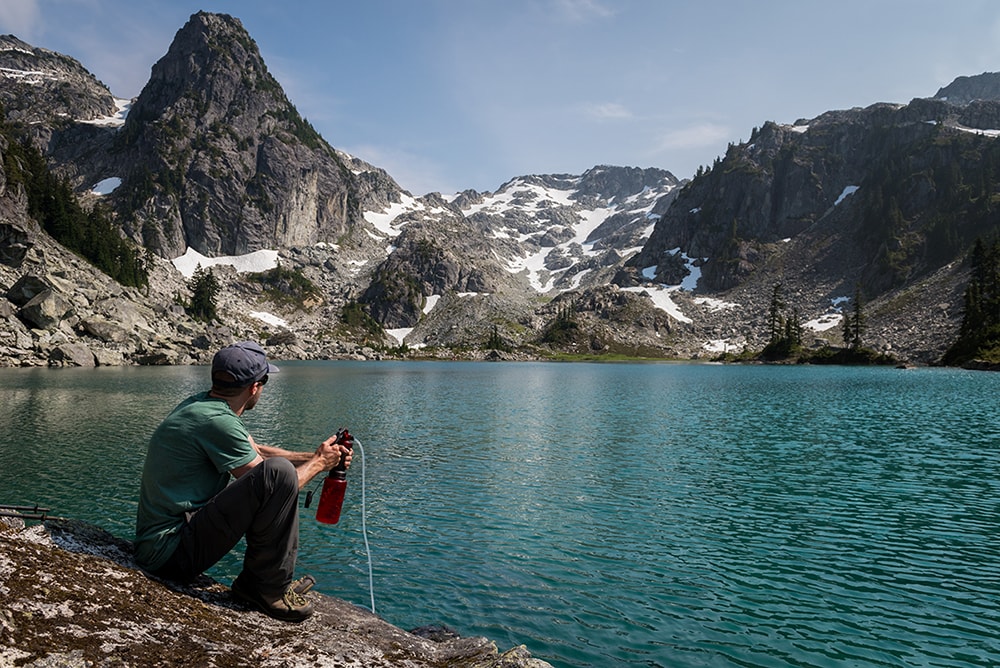In this vibrant outdoor scene, a man is seated at the rocky shore of a serene blue lake, likely nestled at a high elevation, possibly within a volcanic crater. The man wears a dark blue baseball cap, a green short-sleeved t-shirt, gray trousers, and brown hiking boots. He is intently filling his red water bottle via a small white hose dipped into the clear lake water. The setting is bathed in sunlight, highlighting the rocky, vegetation-sparse peaks surrounding the lake, with some patches of snow still visible. Tall mountains rise majestically beyond the lake, with the one on the left featuring a prominent peak. The sky overhead is a crisp blue, adorned with hazy features and scattered white clouds, completing the tranquil and picturesque landscape.